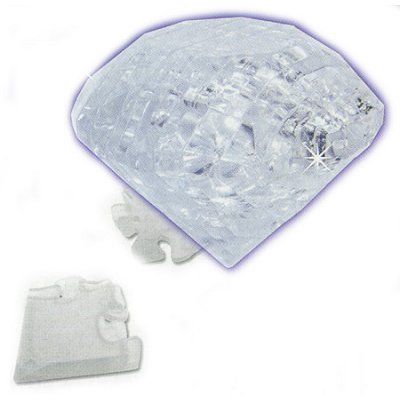The image prominently features a large, silver-white, sparkling crystal that resembles a diamond, positioned slightly towards the upper right corner against a solid white background. The diamond, imposing and textured with a hint of blue on its border, captures the eye with its fake glimmer reflected on its right side, giving it a prestigious and expensive appearance. Occupying about half of the image, this gem's radiance is unmistakable. Two jigsaw puzzle pieces, both translucent and glass-like, are partially visible beneath and to the bottom left of the diamond, with the lower piece likely being two stacked corner pieces with a distinctive protruding shape. The image's meticulous focus on the diamond and the strategic placement of these elements against the minimalist backdrop heightens the overall elegance and grandeur of the composition.